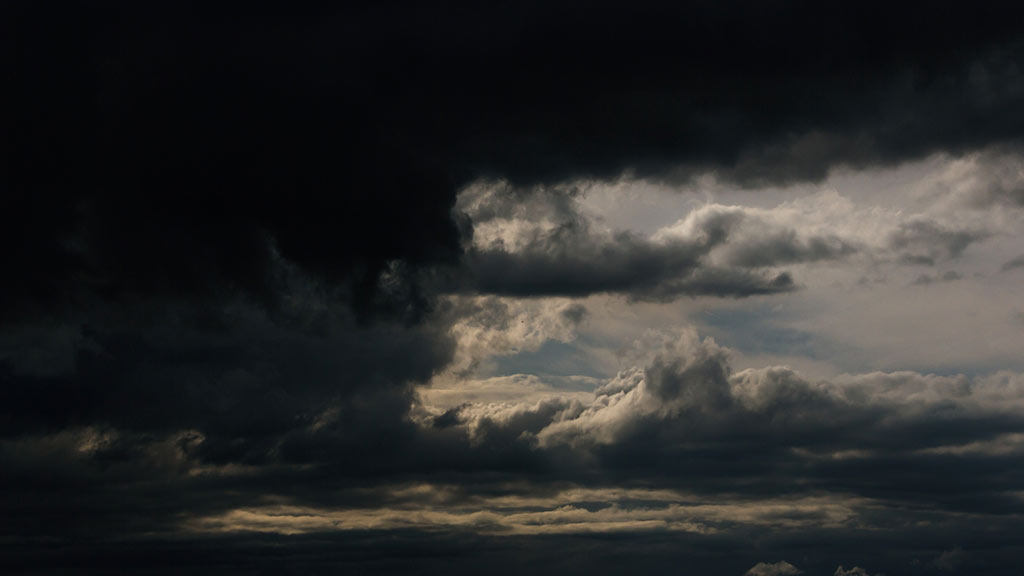The photograph depicts a dramatic sky dominated by a tumultuous mix of clouds. The overwhelming darkness pervades the majority of the frame, particularly on the upper left and outer regions, contributing to a foreboding and ominous atmosphere. Approximately 40 percent of the image is illuminated by a faint light, revealing grayish clouds that appear to be in motion, possibly indicating windy conditions. The faint traces of the horizon or shadowy mountains at the very bottom add to the somber mood. The scene evokes the sense of an impending storm, possibly a hurricane or tornado, with the once-visible blue sky and sunlight now almost entirely obscured by the deep, murky clouds. The overall impression is one of impending doom and environmental upheaval.